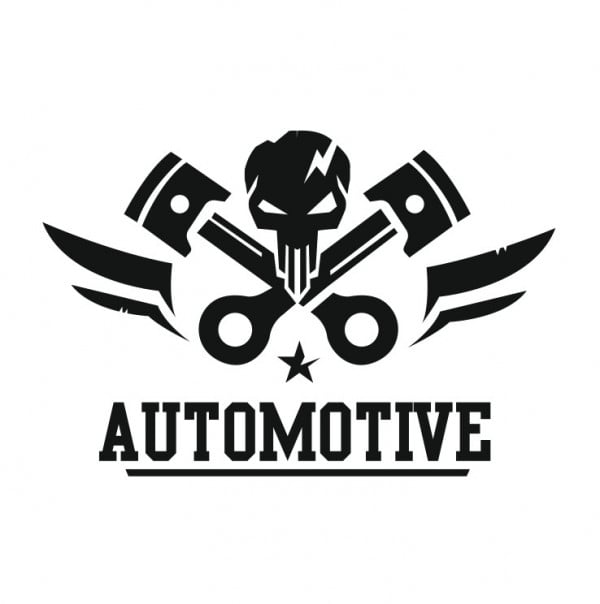The image features a striking black and white logo set against a white background, characterized by several distinct elements. Dominating the center is a skull, distinctively cracked with a lightning bolt running through its middle. Flanking the skull are two crossed structures, which resemble shovels or possibly car parts, adding a unique twist reminiscent of traditional crossed bones. Extending from either side of these crossed elements are wing-like shapes, enhancing the logo's dynamic appearance. Positioned below the skull is a star, slightly unique with one spike featuring a white section. Beneath this star, the word "AUTOMOTIVE" is boldly written in all capital letters and underlined with a horizontal black line, emphasizing the word and tying the design together. This versatile image, suggestive of a sticker, magnet, or digital icon, showcases elements of both mechanical precision and edgy design, making it suitable for various applications.